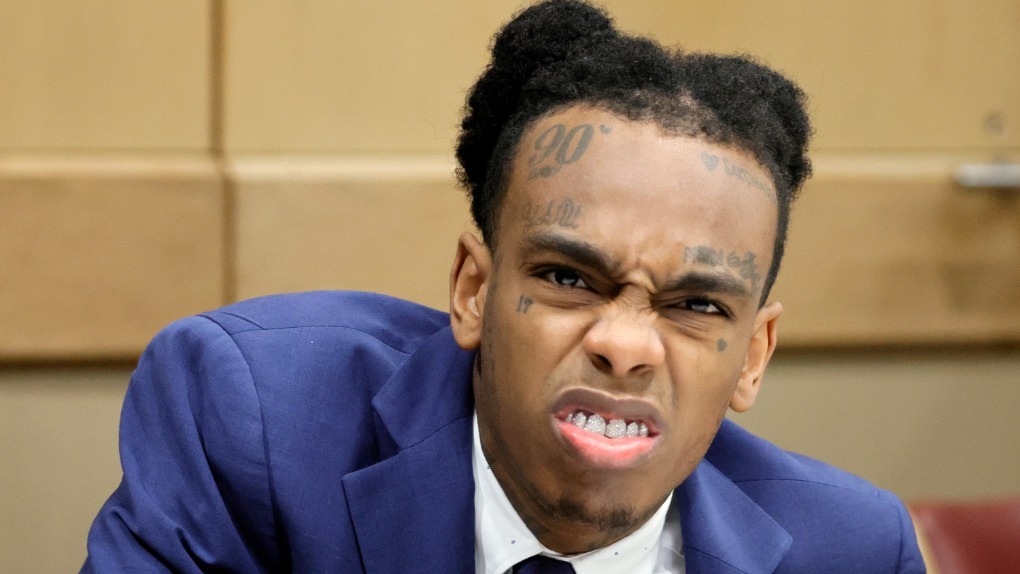The image depicts a close-up of a young African American man, likely in his 20s, who is seemingly reacting to something with a snarl of disgust on his face, revealing his white teeth and wearing a grill. He has matted black hair styled in a way that resembles Mickey Mouse ears atop his head. His face and forehead are extensively tattooed, with notable designs including the number '90', a heart, a tear under his left eye, and the number '17' under his right eye. His expression is one of anger or disapproval, emphasizing his prominent facial tattoos. He is dressed in a blue suit, white shirt, and a tie, although the tie is not very distinguishable. The background features beige, court-like walls, adding context to the setting.